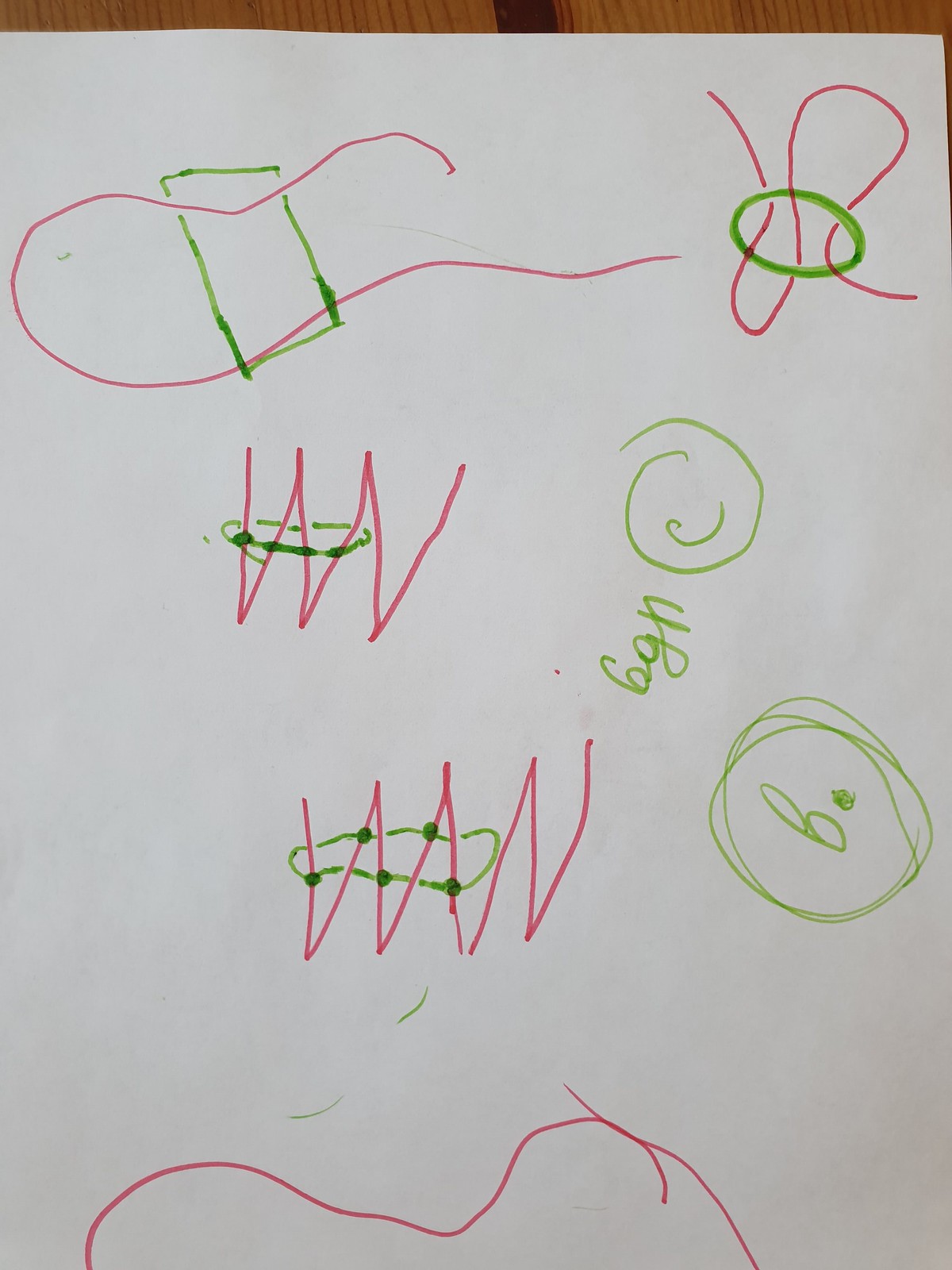Indoor color photograph of a piece of paper adorned with a series of simple doodles executed in pink and lime green. There are approximately six distinct doodles on the page. 

Starting at the upper left, a pink line originates from the middle of the page, arcs slightly diagonally to the left, loops underneath itself, and then returns to the center, ending just a bit to the right. Below this, there is a lime green outline in the shape of a simple rectangle.

To the right of these figures, there is an S-shaped pink line intersected by a green oval, depicting the green oval as if it is looping around the pink line, holding it together.

Lower left and slightly left of center, there is a red W with a V connected to it. Around the left portion of the W, a green circle is drawn.

Right of center, there is a signature in lowercase letters encircled; it reads "BGHC" within a green circle, positioned at a diagonal angle.

At the bottom center, there are two interconnected pink W’s forming a sort of mirrored pattern, enveloped by a green oval that surrounds five vertical lines within the W structures.

To the right of this, there is a pink B encased in three or four concentric green circles.

Finally, at the very bottom, a line starts from the bottom left edge, loops upwards, extends horizontally, shifts slightly diagonally, then loops back down, exiting the bottom edge of the paper.